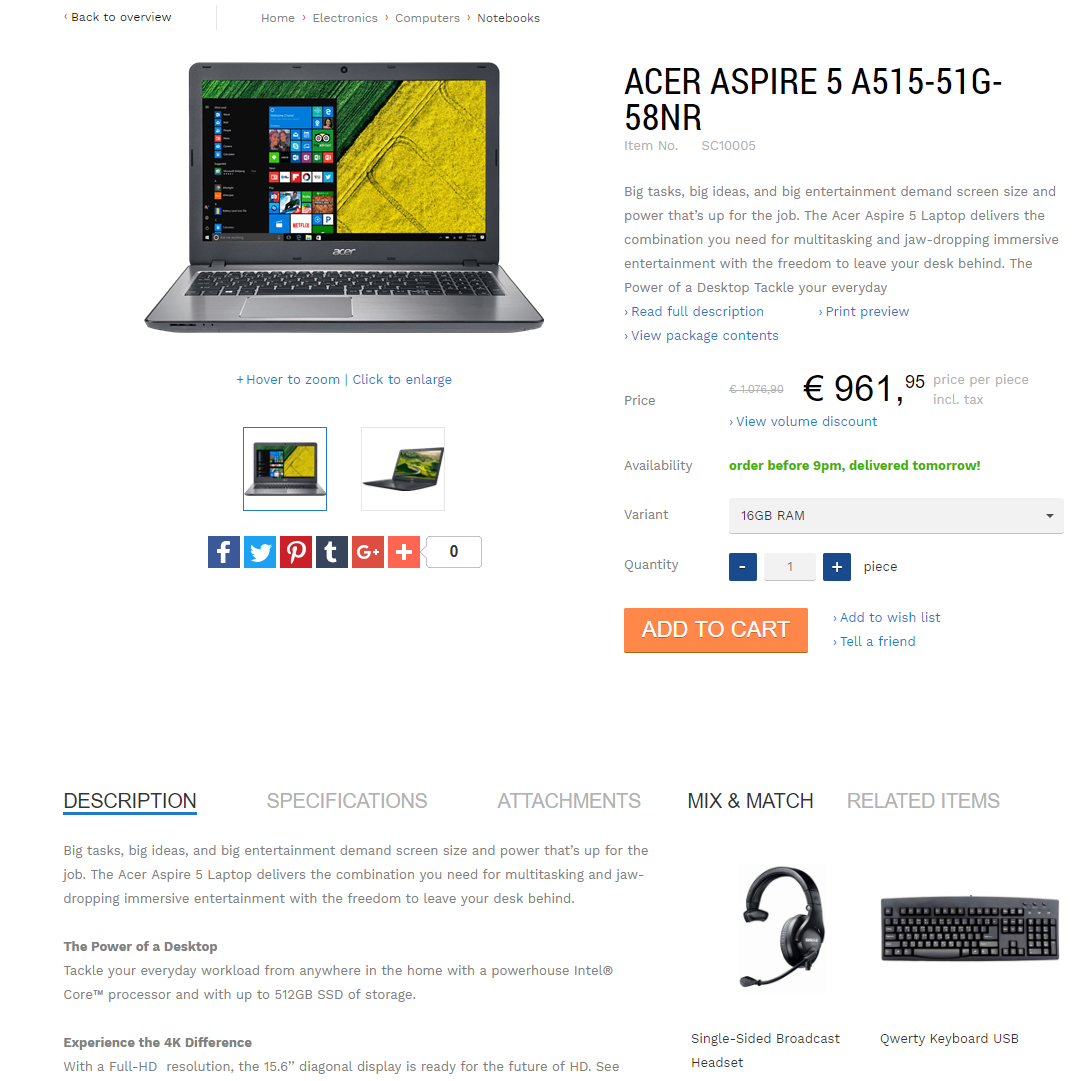The image shows a webpage displaying the Acer Aspire computer on a vibrant background featuring bright colors like pink, blue, and green. The webpage prominently displays the Acer Aspire logo along with the model number and a detailed description of the computer.

The price is listed in Euros as €961.95 per piece, inclusive of tax, and there's an option to view volume discounts. An availability section notes, in green text, that orders placed before 5pm will be delivered by 9pm the next day. Although the layout resembles an Amazon page, no Amazon insignia or branding is visible.

Below the main image of the computer, smaller thumbnail images allow users to view different angles of the device, including the front and side. Social media icons for Facebook, Twitter, Pinterest, and others (T, G, and a plus symbol) are shown beneath the thumbnails, along with a white box displaying the number zero.

Additional sections, labeled as Descriptions, Specifications, Attachments, Mix and Match, and Related Items, provide more detailed information through both text and images about the Acer Aspire computer.